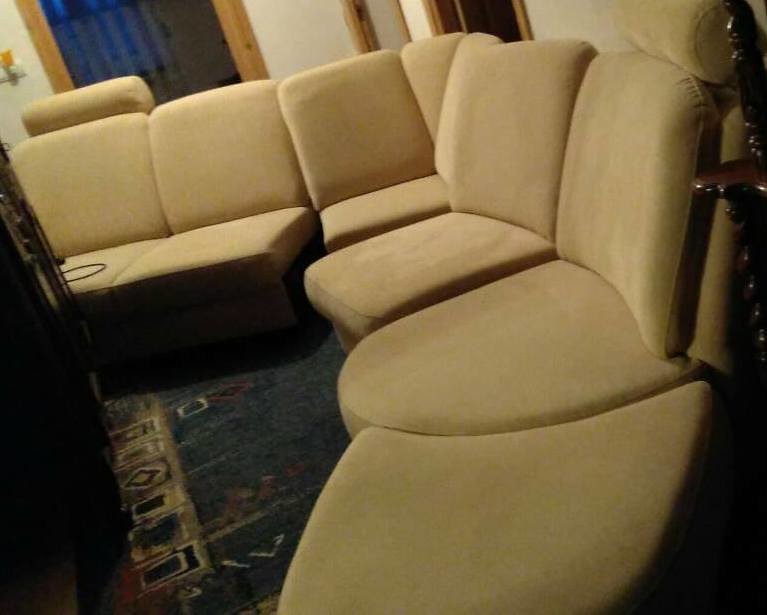In this detailed photograph, a spacious living room is prominently occupied by an L-shaped sectional sofa upholstered in beige fabric. The sectional is composed of multiple pieces, including two joined cushions at the back left, a corner piece slightly separated from them, a single middle piece featuring a rounded center with an adjustable headrest, and another rounded section that appears versatile, possibly serving as an additional seating area or footrest. A dark wooden stand sits to the right of the sectional, adding to the room's functional decor.

The beige sectional boasts accents of shiny dark wood on its frame, enhancing its elegant look. The couch is arranged in an upside-down U shape, facing left, capturing attention with its simple yet sophisticated design.

The living room is furnished with a blue rug that has tan geometric square patterns and a traditional brown wooden side table which appears pillar-like with a flat lighter brown surface. The lighting suggests it's nighttime, with darkness filtering in from an open door at the top left of the image. A sheer curtain partially covers this door, which reveals a dim, starry night outside. Additionally, there's a large black structure resembling a television to the left of the sectional, positioned very close to the couch.

Another door, partially visible on the right, leads to an unseen darkened space, further emphasizing the cozy, enclosed feel of the room. The combination of carefully placed furniture and thoughtful lighting creates a warm, inviting atmosphere in the living area.